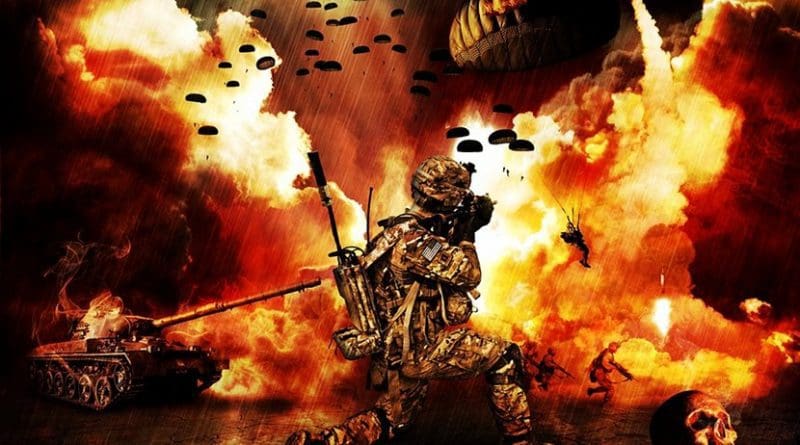In a vibrant and dramatic video game-style illustration, a central warrior figure clad in camouflage kneels on one knee in profile, poised towards the right. The figure appears to be communicating via a walkie-talkie, with a backpack and several weapons visible. This soldier is set against a fiery battlefield dominated by vivid oranges and reds, casting the scene in a dramatic light. In the bottom left, a small, older-model tank erupts in flames, its long barrel directed to the right. To the tank’s right lies a partially visible skull and a cluster of soldiers sprinting in the background. The sky above is dotted with approximately 15 to 20 paratroopers descending amidst the chaos, some silhouetted against the inferno. The intense explosions illuminate the scene, contrasting starkly with the darkened areas outside the fiery ground zero, emphasizing the explosive destruction below.